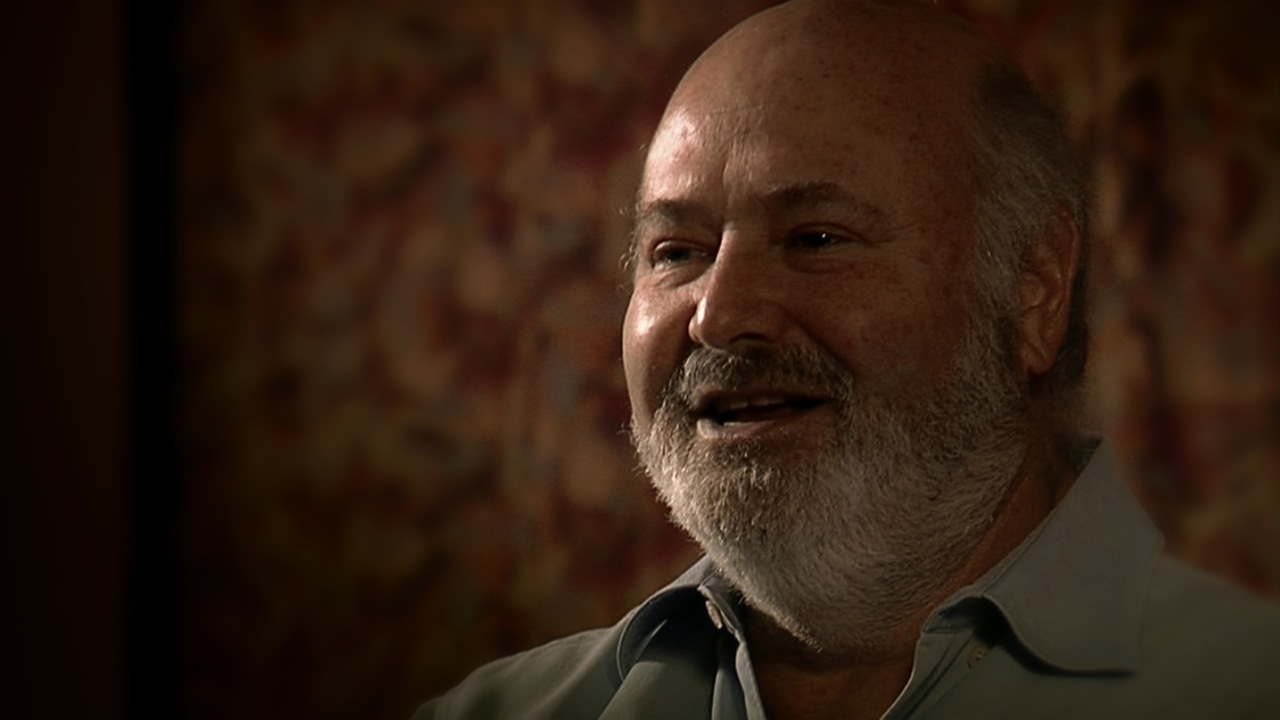The image captures Rob Reiner, the esteemed actor and director, now with gray hair, a white beard, and notably balding, speaking and smiling. Dressed in an olive green collared shirt, he sits on the right side of the photograph, with his mouth slightly open as if mid-conversation. The setting is a dimly lit room, casting shadows that highlight the left side of his face. The background is a blurred mixture of red, white, purple, and yellow hues that suggests an art piece, decorative wall, or possibly an oriental rug. The setting appears intimate, focusing on Reiner's expressive demeanor while he engages in what seems to be an amiable dialogue.